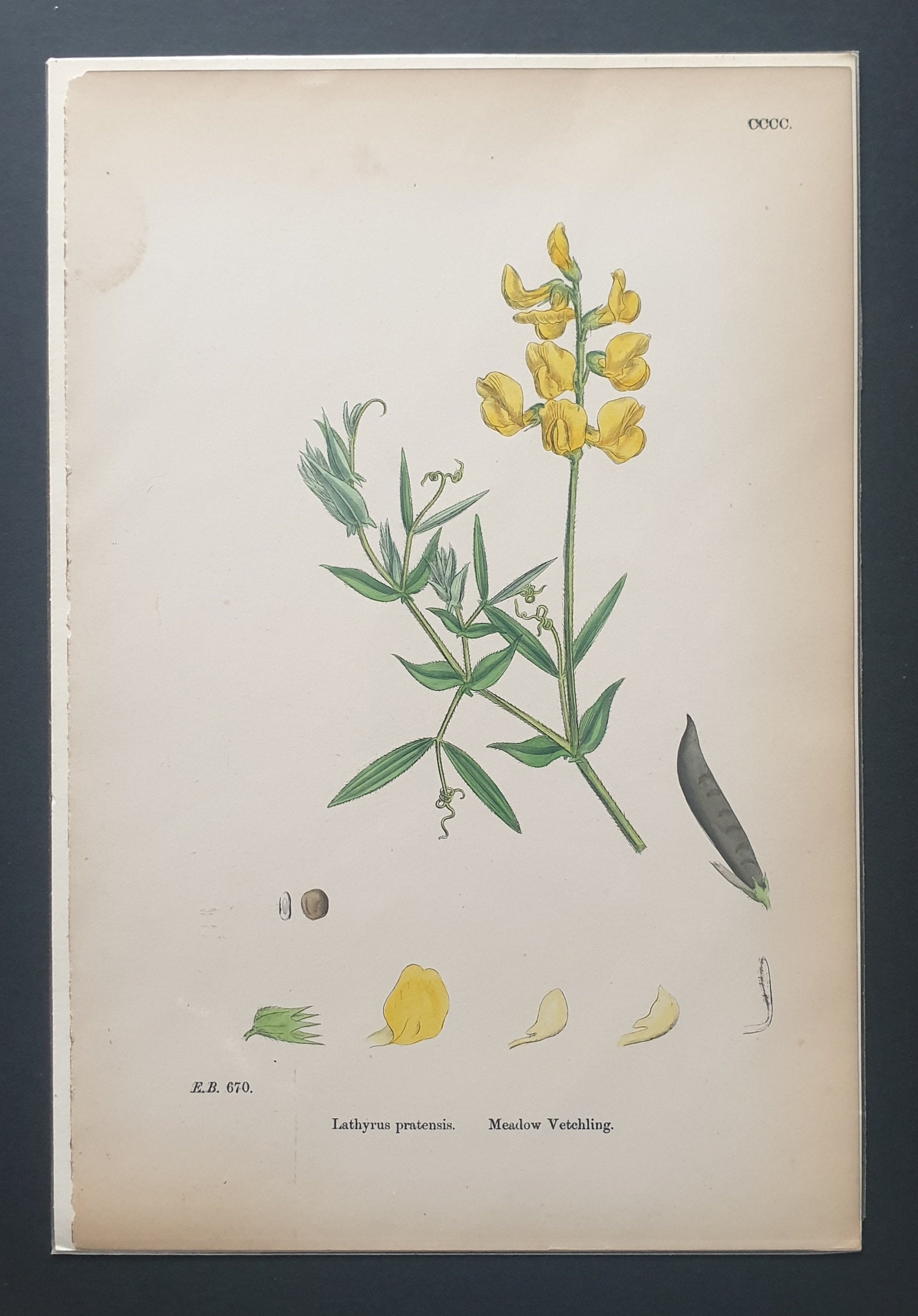The vertically aligned, framed image resembles an artistic painting of a flower. The frame is a thick, charcoal-colored border, nearly black, that encloses a background of aged beige paper, exhibiting brown stains, particularly in the upper left area. The centerpiece of the image is a green stem adorned with green leaves and topped with yellow flower petals, visually reflecting the flower species Lathyrus pratensis. Below the main flower illustration, the image displays a detailed deconstruction of the flower's components, laid out horizontally: on the left is a single leaf, next to it a yellow petal, followed by two smaller yellow petals labeled as "Meadow Vetchling." Additionally, there is an illustration of a black pea pod-like structure on the right. The background paper shows signs of aging, with browning edges and wear. A small legend at the bottom includes the names "Lathyrus pretensis" and "Meadow Vetchling," along with a notation "EB670".